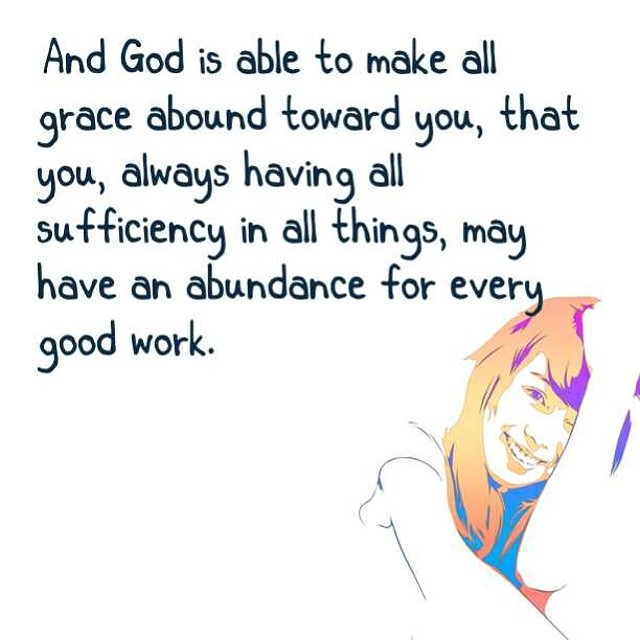The image features an inspirational quote on a white background. The main focal point is a biblical verse in dark blue, almost black letters that reads, "And God is able to make all grace abound toward you; that you, always having all sufficiency in all things, may have an abundance for every good work." This text is arranged into six lines and is positioned towards the top left corner of the image.

In the bottom right corner, there is a detailed, partially outlined artistic drawing of a young girl. Her hair is a vibrant mix of yellow, orange, purple, and blue hues. She is wearing a short-sleeved shirt, likely blue, and is smiling with her head tilted to her left. One of her eyes is closed, and the other is colored purple. Her forearm is covering part of her face. The colors used in the illustration are very saturated and include shades of blue, yellow, and purple, but her arms remain uncolored. There are no other persons, animals, or artistic elements in the picture.

Overall, the primary colors in the image are blue, yellow, and black, contributing to a harmonious yet vivid feel that emphasizes the inspirational message.